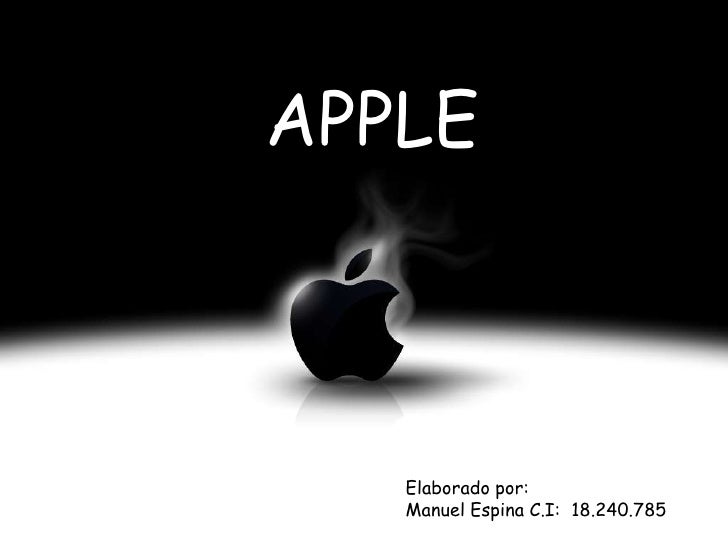This is a digitally created black and white image featuring the iconic Apple logo at its center. The black Apple logo, complete with its traditional bite taken out, sits on a reflective white circular surface. Above it, in uppercase white letters resembling a kindergarten font, the word "Apple" is prominently displayed. A light source shines on the left side of the logo, while a mist or smoke emanates from behind, creating a foggy effect against the otherwise black background. Below the logo, towards the bottom right corner, the text in black reads: "elaborado por Manuel Espina CI 18.240.785," indicating the creator's details in Spanish. The overall composition highlights a stark contrast between the black Apple logo and the vivid white elements, emphasizing its distinct and familiar design.